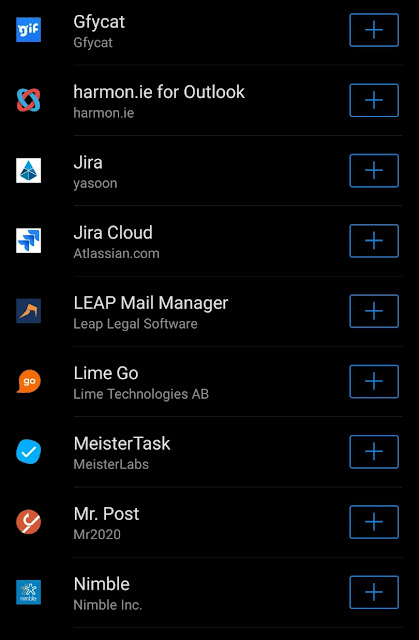Screenshot of a smartphone showing a list of apps set against a pitch-black background. The screen is oriented in portrait mode. The left side features a vertical column of icons with labels next to them. The topmost icon is labeled "GFY Cat." A series of identical icons, each accompanied by blue-bordered rectangles containing blue plus signs, run down the left side. Below, the following app names are sequentially listed: "Harmon.ie for Outlook," "Harmon.ie," "Jira," "Yassoon," "Jira Cloud," "Leap Mail Manager," "Line Go," "Meister Task," "Mr. Post," and "Nimble." The list ends at the bottom of the screen. Each app name is neatly aligned, with smaller font subtitles where noted.